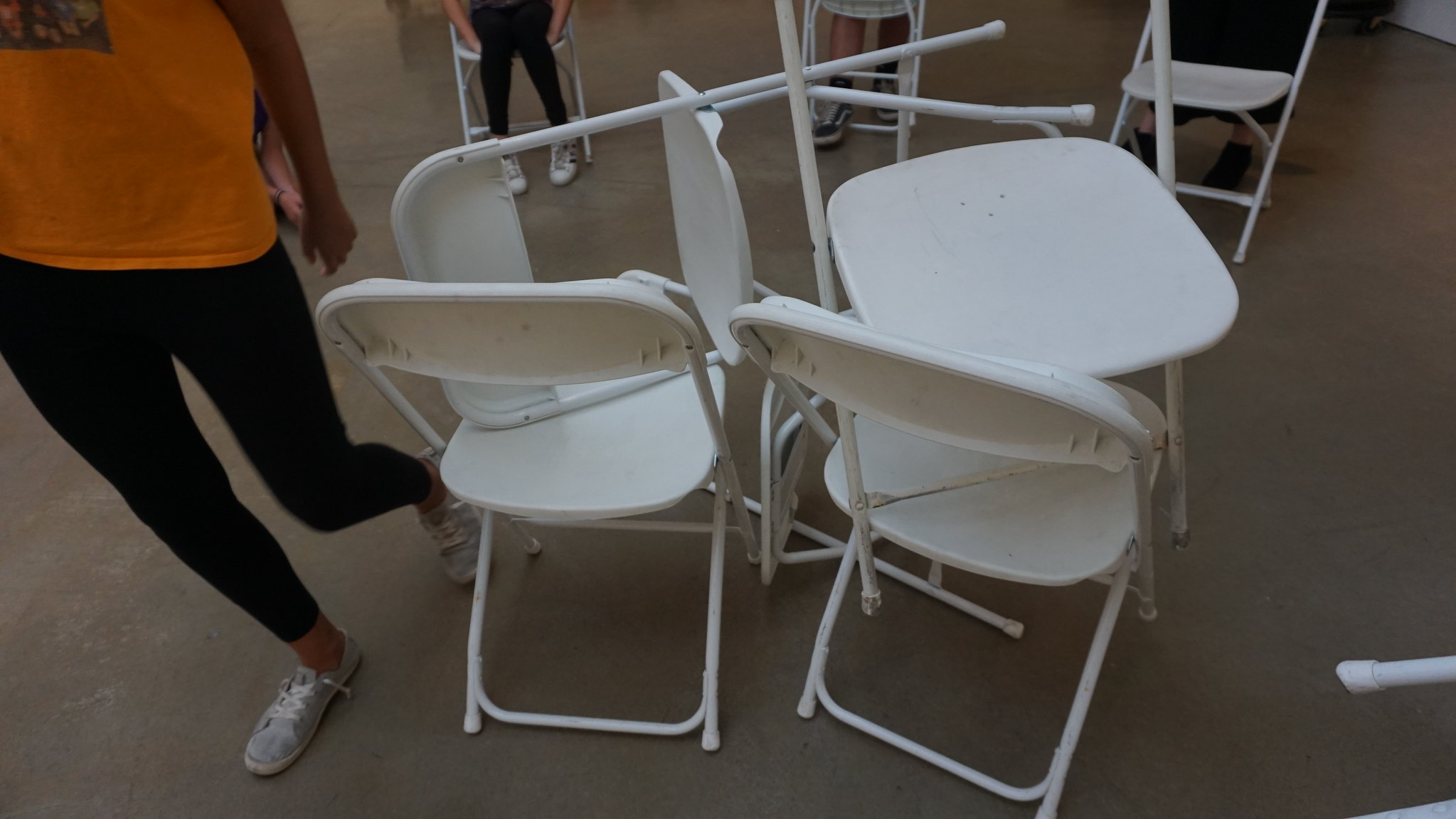The image captures a chaotic arrangement of white steel folding chairs, some stacked haphazardly. Two chairs stand on their legs, supporting another two chairs lying on top in various positions—one on its side and the other inverted. The scene suggests either a cleanup process or preparation for an event. In the foreground, to the left, stands a woman—slim, with light skin—dressed in black, skin-tight leggings, white tennis shoes, and an orange-yellow shirt that features a graphic, although it's mostly obscured. Her arm is extended at her side. In the background, several other white chairs are occupied. One person in black leggings sits with her hands underneath her legs, while another pair of gray sneakers is visible. A third person stands behind a chair to the right. The environment appears industrial, with a dark gray or tan stone-like floor, adding to the overall utilitarian atmosphere.